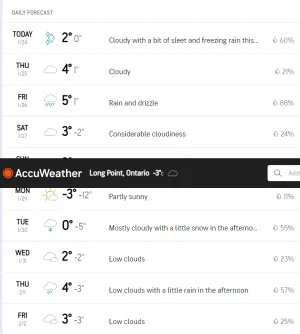This close-up screenshot captures detailed weather information from a website or application, featuring a predominantly white background. A thin gray vertical line runs along the left side of the image, immediately drawing the viewer’s eye. At the top left, the label "DAILY FORECAST" is presented in light gray, all-caps, sans-serif text, followed by a thin gray line that separates it from the rows of weather details below.

These rows are arranged neatly with thin gray dividing lines between them. Positioned centrally, there is an overlay spanning two rows with a dark gray background. On the left side of the overlay, a red sun icon is displayed next to the white text "ACCUWEATHER". Following this, smaller white text reads "LONGPOINT, ONTARIO, -3°C", and to the very right of this text, there's a light gray cloud icon.

Towards the right side of the overlay, there is a partially visible search bar, truncated by the edge of the frame. Each row begins with the day of the week, starting with "TODAY" in black text, followed by "THURSDAY", and continuing in succession. Directly beneath "TODAY", in light gray text, is the date "1-24".

Further to the right of each day's label, there is an icon indicating the weather conditions for that day. Adjacent to the icon, the forecasted temperature is displayed in larger black numbers, with a smaller degree value in medium gray next to it. Following some negative space, a brief description of the day's weather is provided in black text. For instance, "TODAY" is noted as "CLOUDY WITH A BIT OF SLEET AND FREEZING RAIN...". Finally, a light gray raindrop icon with a percentage value appears at the far right, indicating the probability of precipitation for the day.